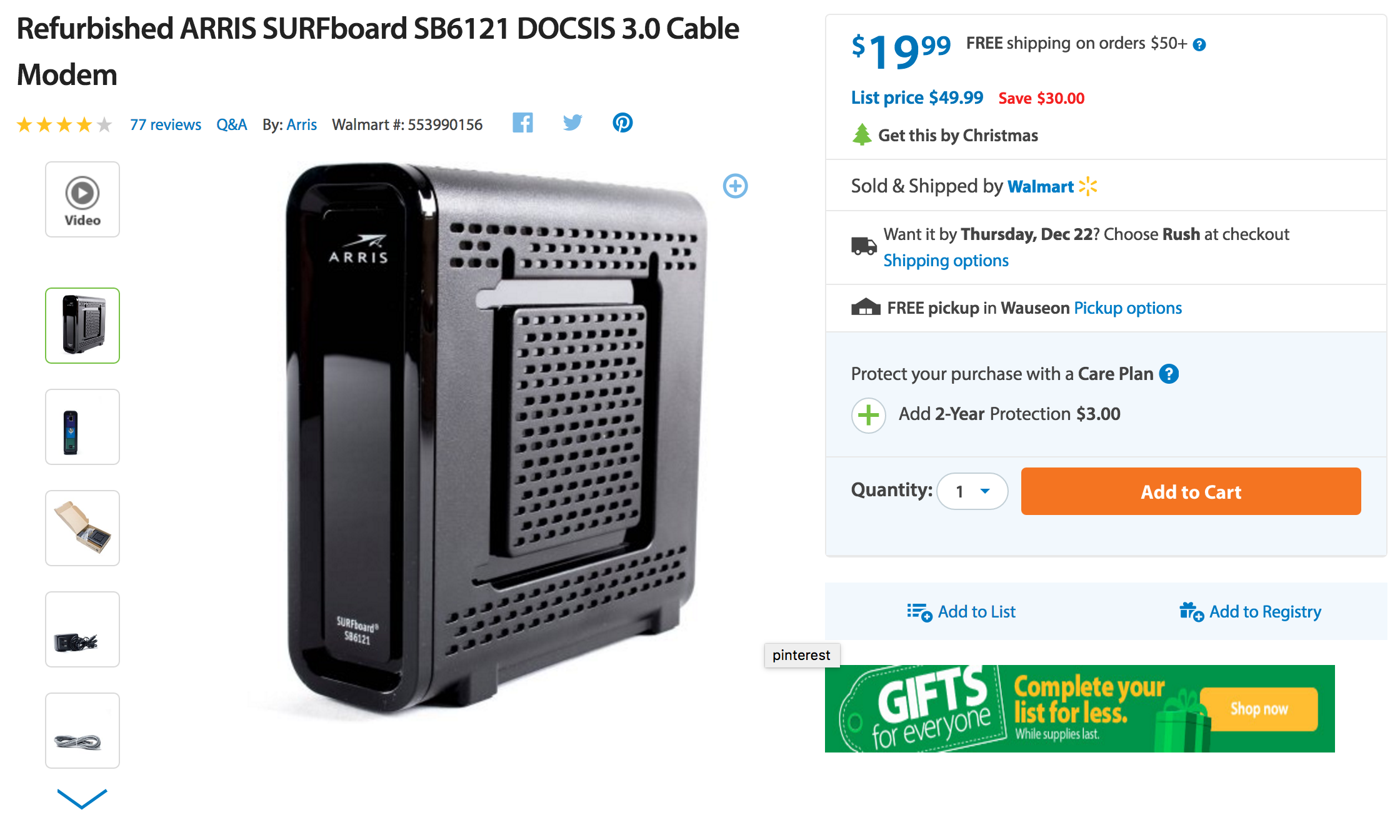This image showcases a refurbished ARRIS SURFboard SB6121 DOCSIS 3.0 Cable Modem, available for purchase on the Walmart website. The modem has received a rating of four stars based on 77 customer reviews. Detailed information includes the manufacturer, ARRIS, along with the Walmart SKU number 553990156.

Special offers include free shipping on orders priced at $19.99, providing a saving of $30 from the original list price of $49.99, bringing the modem's current price to $19.99. The promotion also highlights the possibility of receiving the item by Christmas. Additionally, customers have the option to add a two-year protection plan for $3. The image also features a section to select the item quantity, which is preset to one, along with an 'Add to Cart' button for easy purchasing.